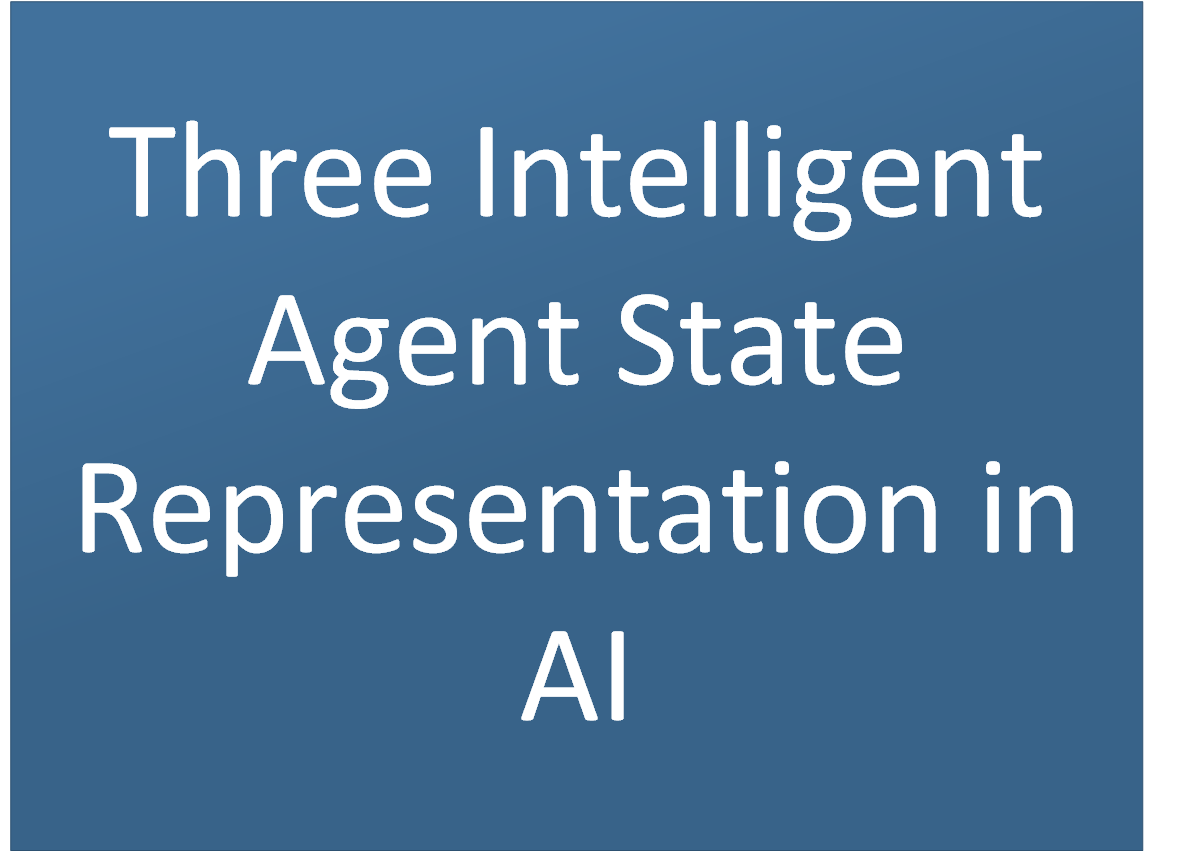The image features a solid bluish rectangle background with no visible specks or additional elements. Overlaid on this background are four rows of bold, white text in capital letters. The text is as follows:

1. "THREE"
2. "INTELLIGENT AGENT"
3. "STATE REPRESENTATION"
4. "IN AI"

The wording appears in a clean, professional font, possibly created using presentation software such as PowerPoint or Canva. The phrase "Three Intelligent Agent State Representation in AI" suggests that the content of the image may be related to a seminar or presentation on the topic of artificial intelligence, focusing specifically on the concept of intelligent agents and their state representation.